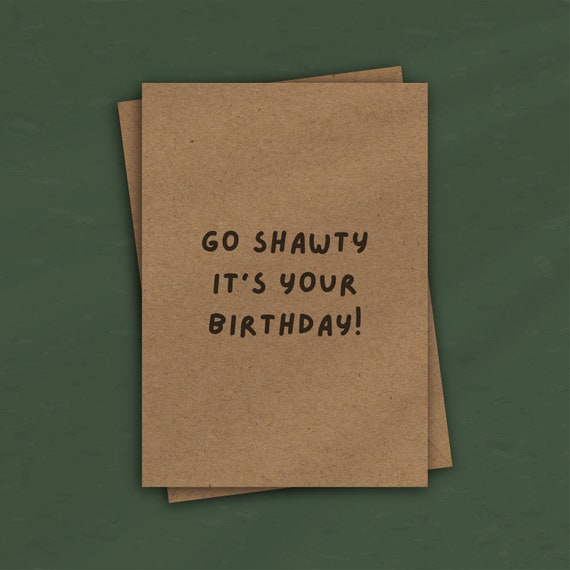This image showcases two pieces of light brown, smooth cardboard or paper bag material, stacked atop each other on an olive or avocado-green background, which may be a table or simply an uncluttered surface. The top piece features black text in all capital letters reading, "GO SHAWTY! IT'S YOUR BIRTHDAY!" with an exclamation point. The underlying piece of cardboard, slightly tilted and identical in size, peeks out along the edges. The overall scene carries a minimalist aesthetic with a faint reflection hinting at a light source, adding a subtle depth to the image.